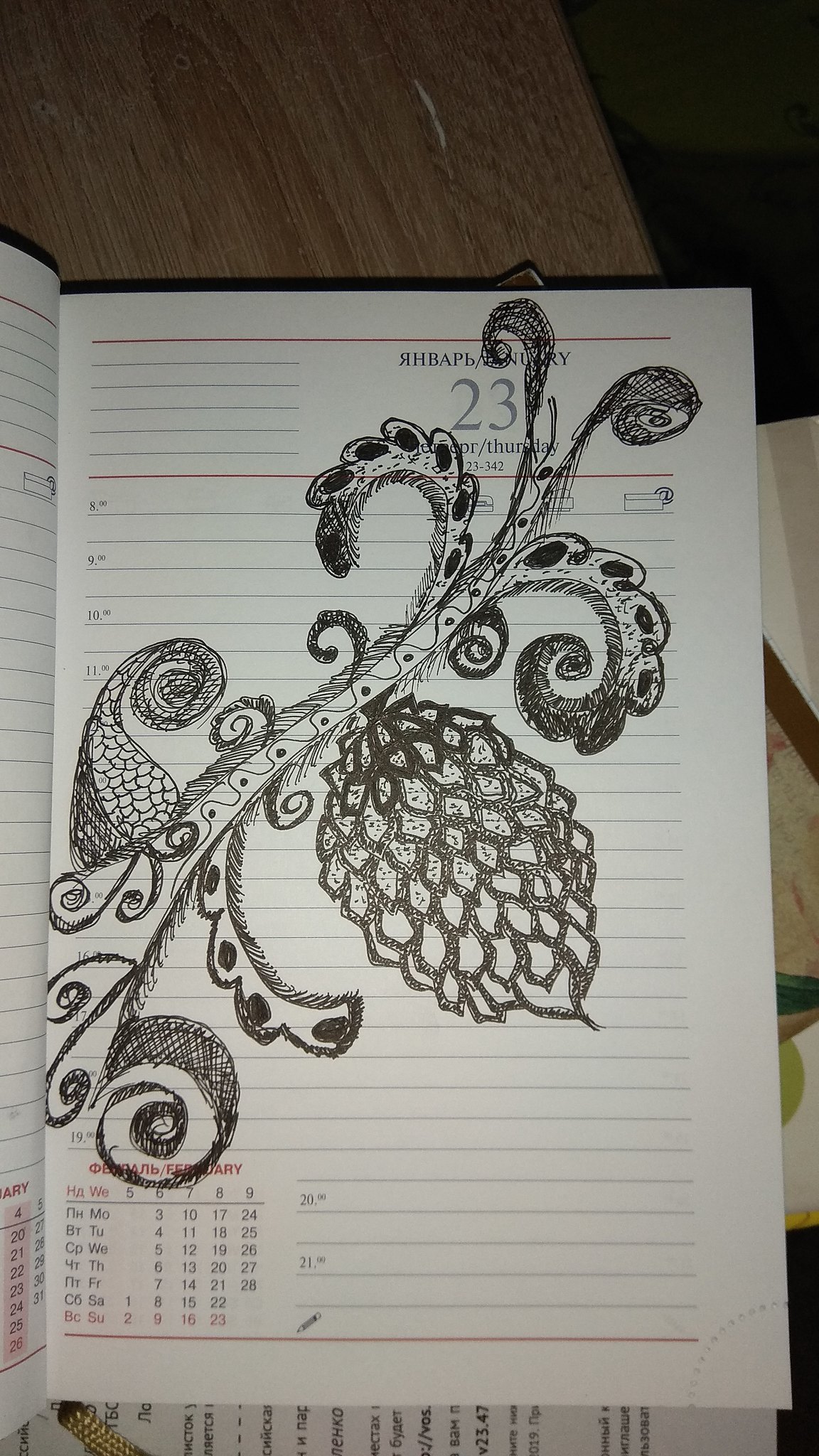The image depicts an open day planner or calendar, placed flat on a medium-brown wooden table with visible wood grain patterns and a small white scratch. The planner has a black border and white pages with a mix of black, grey, and red text. The left bottom corner of the page showcases the days of the week in what appears to be Cyrillic or Russian, including the number 23 and the word "Thursday."

Inside the planner is a detailed black pen illustration of a plant. The drawing features intricate, curly vines spreading out elegantly, with various leaves stemming from the main branches. Towards the bottom, there is a prominent, larger shape resembling an acorn made up of clustered, harder-edged forms. Overlapping the planner are additional white papers, and a pen or pencil is partially visible. The entire scene is captured from a top-down perspective, emphasizing the artistic intricacies of the plant against the structured layout of the planner.